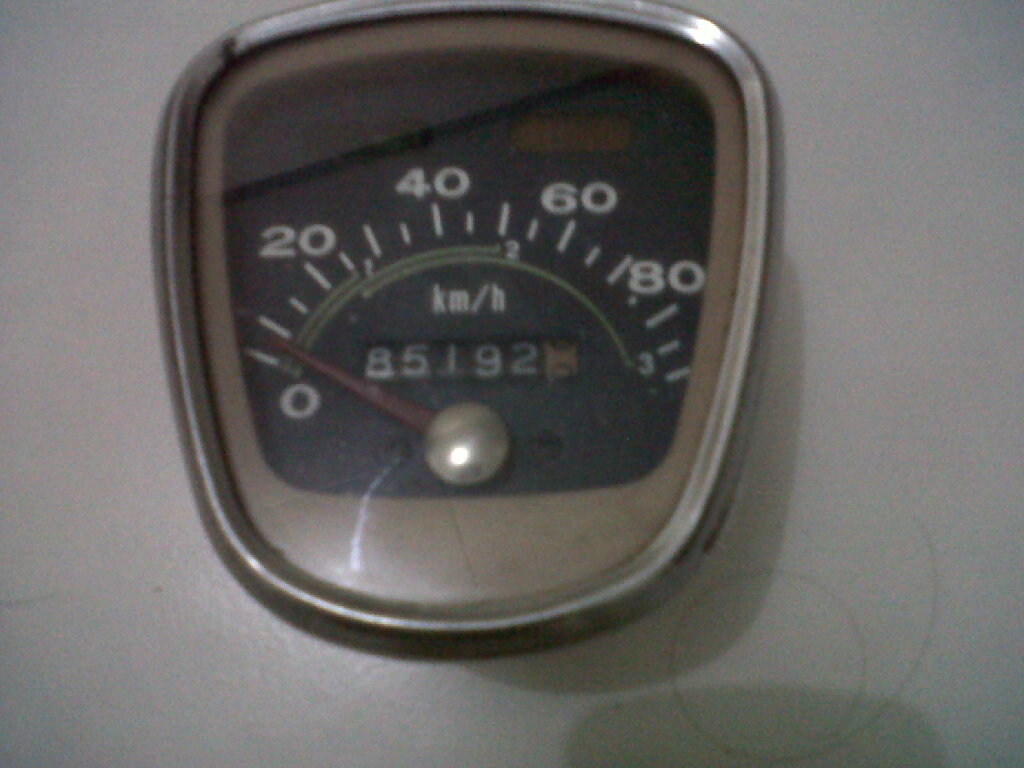The image presents a detailed view of a speedometer set against a gray background. Dominating the center, the speedometer features a circular, black dial encased in a glass cover. This dial is marked in increments: 0, 20, 40, 60, and 80 kilometers per hour are highlighted with thicker lines, and the gaps between these numbers are divided into smaller increments of 5 km/h with thinner dashes. Additionally, green lines run across the dial, further indicating 1, 2, and 3 km/h measurements.

Surrounding the speedometer face, there's a mixture of white and brown elements, with brown headwinds creating a dynamic look. The display shows a mileage indicator reading "8512" along with a small grayish-silver dot, with a hint of red visible on the left side. On the bottom right of the speedometer, there is a circular element framed in white.

Notably, at the top left and top right of the speedometer, there are sections intended for additional information, possibly text. However, in this image, those sections are not illuminated.

The intricate design and fine detailing of the speedometer, from the precise dashes between increments to the small, colored accents, make this image a comprehensive depiction of a classic automotive instrument panel.